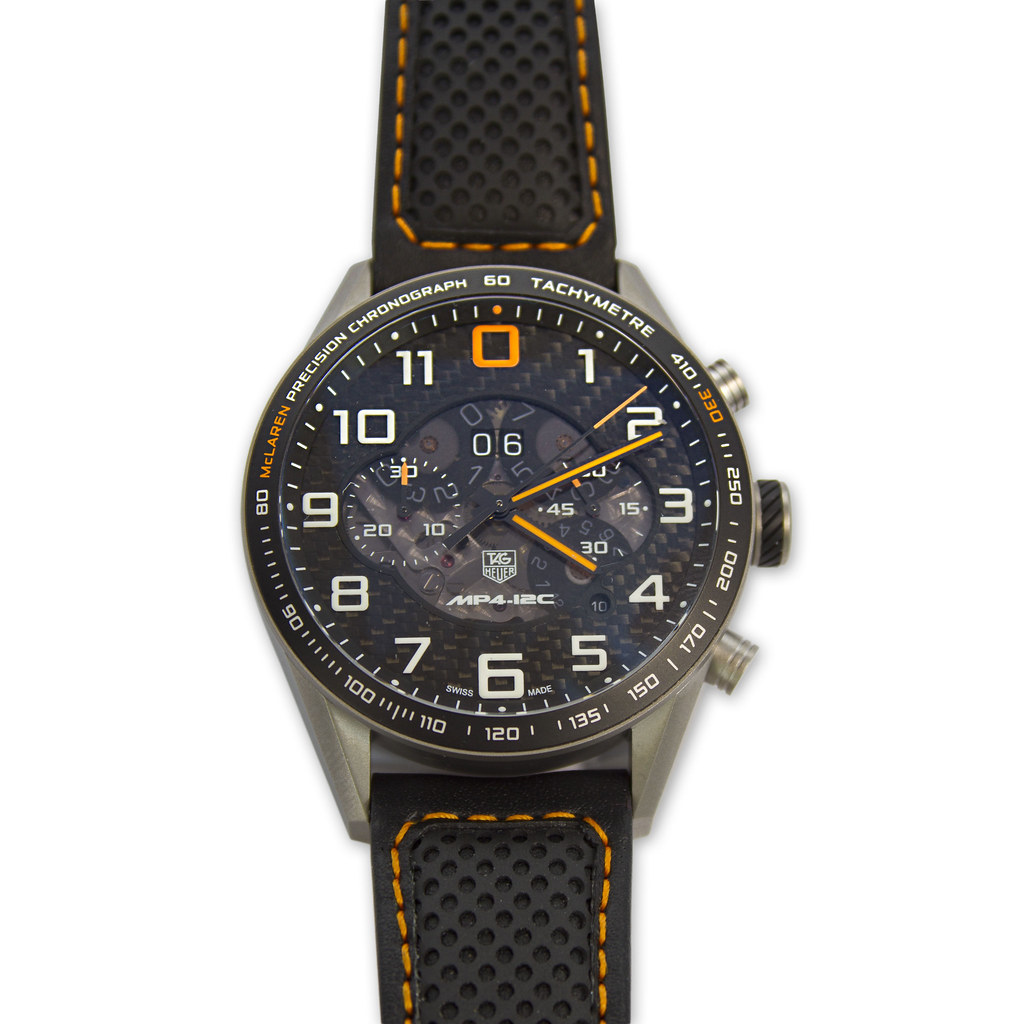The image displays a close-up of a TAG Heuer sports watch against a completely white background. The watch features a black rubber strap with distinctive orange stitching running along the center, accentuated by a textured grip. The watch's case is a combination of black and silver, transitioning from the black strap and grip into a light silver at the connection point, with a true silver finish banding the main head of the watch. 

The watch face is predominantly black, with white numerals for hours, except for the 12 which is replaced by an orange zero. The hands of the watch—minute, hour, and second—are black with orange stripes. The text "TAG Heuer" and the logo are prominently displayed in the center. The watch displays additional details, including "Precision Chronograph," "tachymeter," and numbers such as 410, 330, and 250 around the dial. Additionally, the outer rim displays markings starting from 60 at the top and continues around the face.

Three buttons or knobs on the right allow for adjustment, and a small window reveals the watch's intricate internal gears, with additional white numbering for precise timekeeping. The face also features a separate sub-dial with numbers like 10, 20, and 30, and a digital display showing "06". Orange text spelling "McLaren" highlights the partnership branding, underscoring this watch's sporty, precise, and luxurious design.